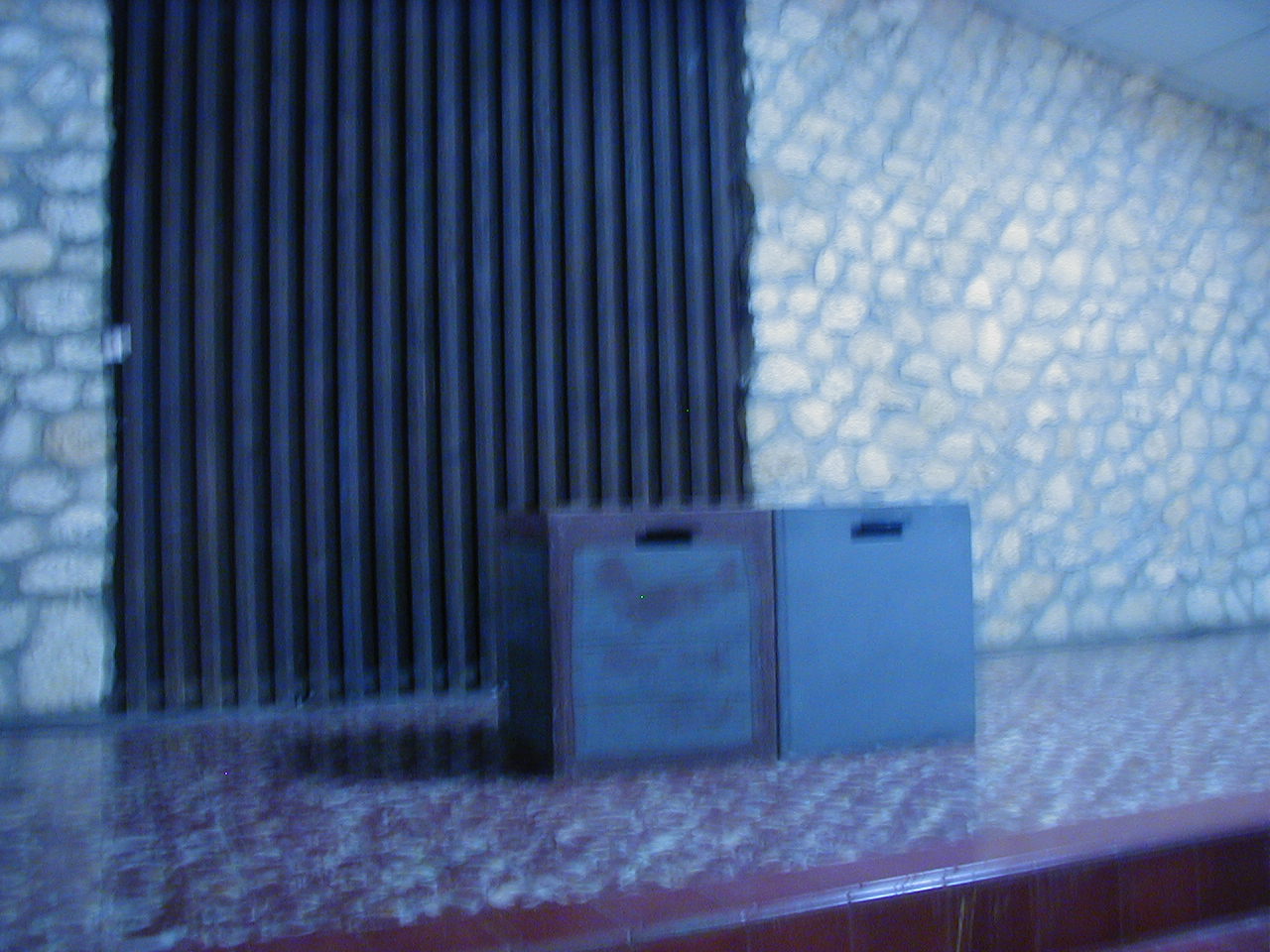This extremely blurry photograph appears to capture an elevated surface that resembles a stage or countertop, characterized by maroon and white marbled tiles. The front edge of this elevated surface steps up from the lower floor and is bordered with solid red tiles. Upon this surface rest two crates in close proximity: the crate on the left is gray and red with purplish-blue designs and handles for carrying, while the crate on the right is a solid gray with similar handle cutouts. In the background, the wall is composed of rounded white and gray stones, with dark vertical slats—likely metal—flanking a silver-latched metal sheet door on the left. The ceiling features white dropdown panels, rounding out what appears to be a formal setting, possibly a church or business. Despite the blurriness suggesting a motion-captured shot, the overall staging hints at a meticulous, structured environment.